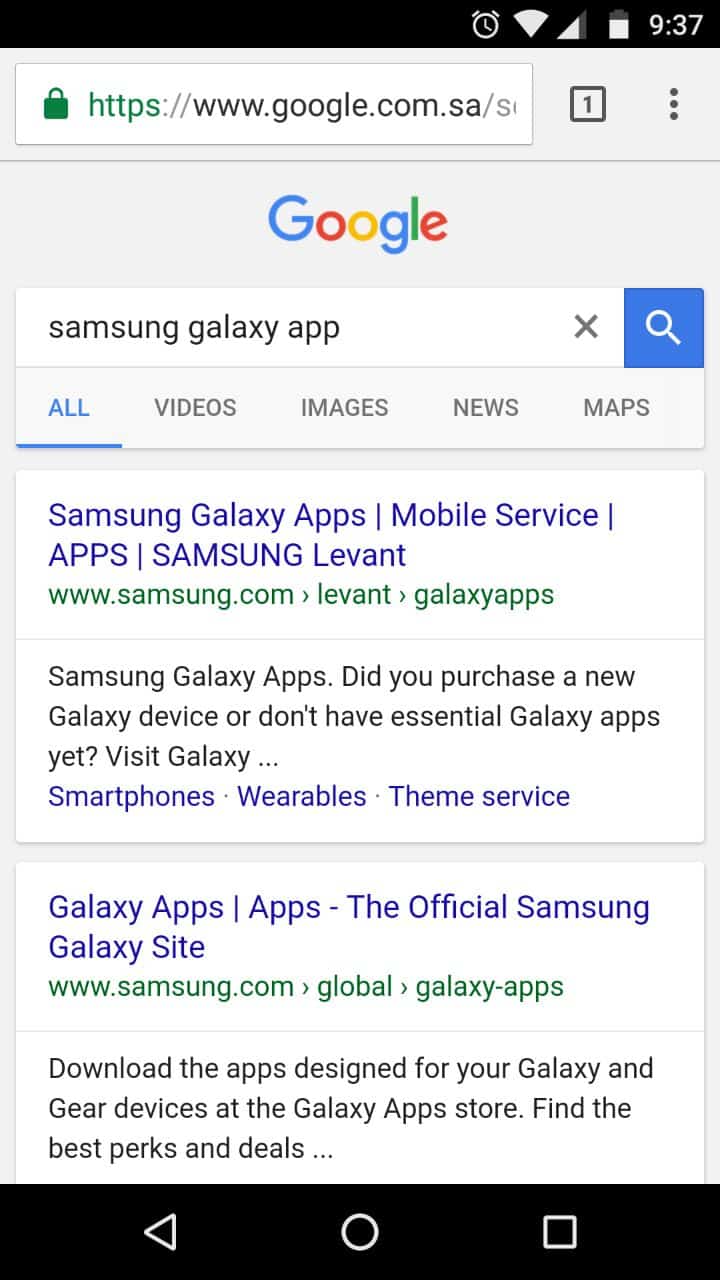Screenshot of Google search results for 'Samsung Galaxy app' showing various informational elements. The top of the page displays the Google logo prominently beside the search bar, which contains the entered query, 'Samsung Galaxy app'. To the right of the text entry, there is an 'X' icon for clearing the search, followed by a blue box with a white magnifying glass icon, indicating the search button.

Directly below the search bar, there is a navigation line featuring options: All, Videos, Images, News, and App. The 'All' option is selected and highlighted in blue with a corresponding blue underline.

The search results are displayed in boxed snippets below. The first box includes headings and descriptions from Samsung's website, such as:
- Samsung Galaxy apps, mobile service apps, Samsung Levant, Samsung.com, Levant (with an arrow pointing to the right).
- Descriptive text about the availability and benefits of Samsung Galaxy apps, suggesting a visit to the Galaxy apps page for essential services and apps for smart phones, wearables, and themes.

The second result box reads:
- Galaxy apps, line, app, stash, the official Samsung Galaxy site, Samsung.com, (with an arrow pointing to the right), global (with an arrow pointing to the right), Galaxy apps.
- It provides a description encouraging users to download apps designed for Galaxy and Gear devices from the Galaxy Apps store, emphasizing finding the best personal deals.

In the top right corner of the image, the time is displayed as 9:37. The background of the page is white, while a black bar appears at the bottom of the image featuring navigation icons: an arrow pointing to the left, a circle, and a square.